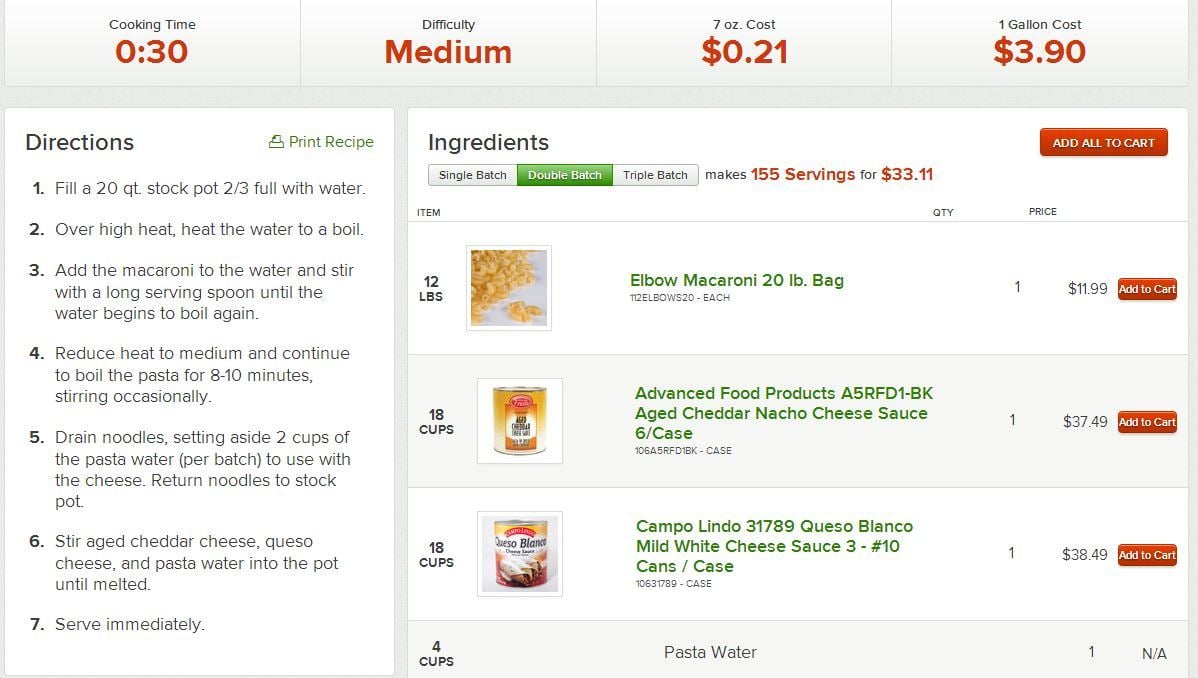### Descriptive Image Caption

**Top Section:**
- **Background:** Gray with black overlay.
- **Text Details:**
  - "Click in Time" in red.
  - "0:30" in black, indicating a time of 30 minutes.
  - "Difficulty" in black with "Medium" in red.

**Middle Section:**
- **Costs:**
  - "7 oz" in black with corresponding cost "$0.21" in red.
  - "1 gallon" in black with corresponding cost "$3.90" in red.

**Left-Side Directions Box:**
- **White Rectangle with Instructions in Black:**
  1. Fill a 20-quart stock pot two-thirds full with water.
  2. Heat the water over high heat until it begins to boil.
  3. Add the macaroni to the boiling water and stir with a long serving spoon until the water resumes boiling.
  4. Reduce heat to medium and continue boiling the pasta for 8 to 10 minutes, stirring occasionally.
  5. Drain the noodles, setting aside 2 cups of pasta water for the cheese sauce, then return noodles to the stock pot.
  6. Stir in eggs, cheddar cheese, queso cheese, and pasta water until fully melted.
  7. Serve immediately.

**Upper Right Section:**
- **Text Details:**
  - "Ingredient Print Recipe" in black.
  - "Ingredients" in black.

**Ingredients List (in green):**
- Elbow macaroni (20 lb bag)
- Advanced Food Products aged cheddar nacho cheese sauce
- Campo Lindo queso blanco mild white cheese sauce